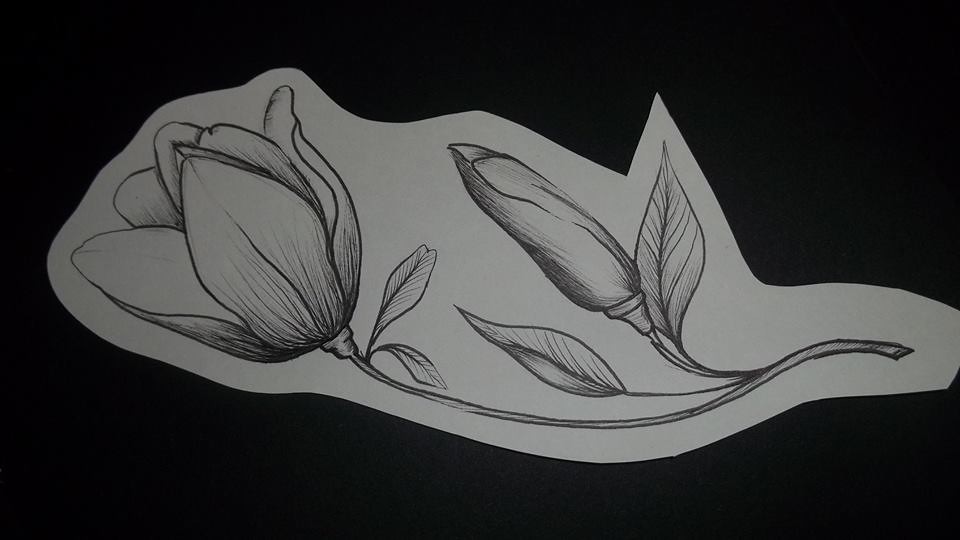This pencil drawing features two distinct flowers rendered entirely in black and white. The larger flower, situated above, showcases multiple blooms accompanied by a variety of leaves, adding to its intricate appearance. Below it, a smaller flower appears with three narrow leaves, contributing to its more delicate and streamlined form. Both flowers are connected by a single vine, creating a unified composition. The artwork is displayed on a uniquely shaped piece of paper, akin to construction paper, which stands out against a contrasting black background. This artistic piece could easily serve as an elegant element in a school project or a creative endeavor.